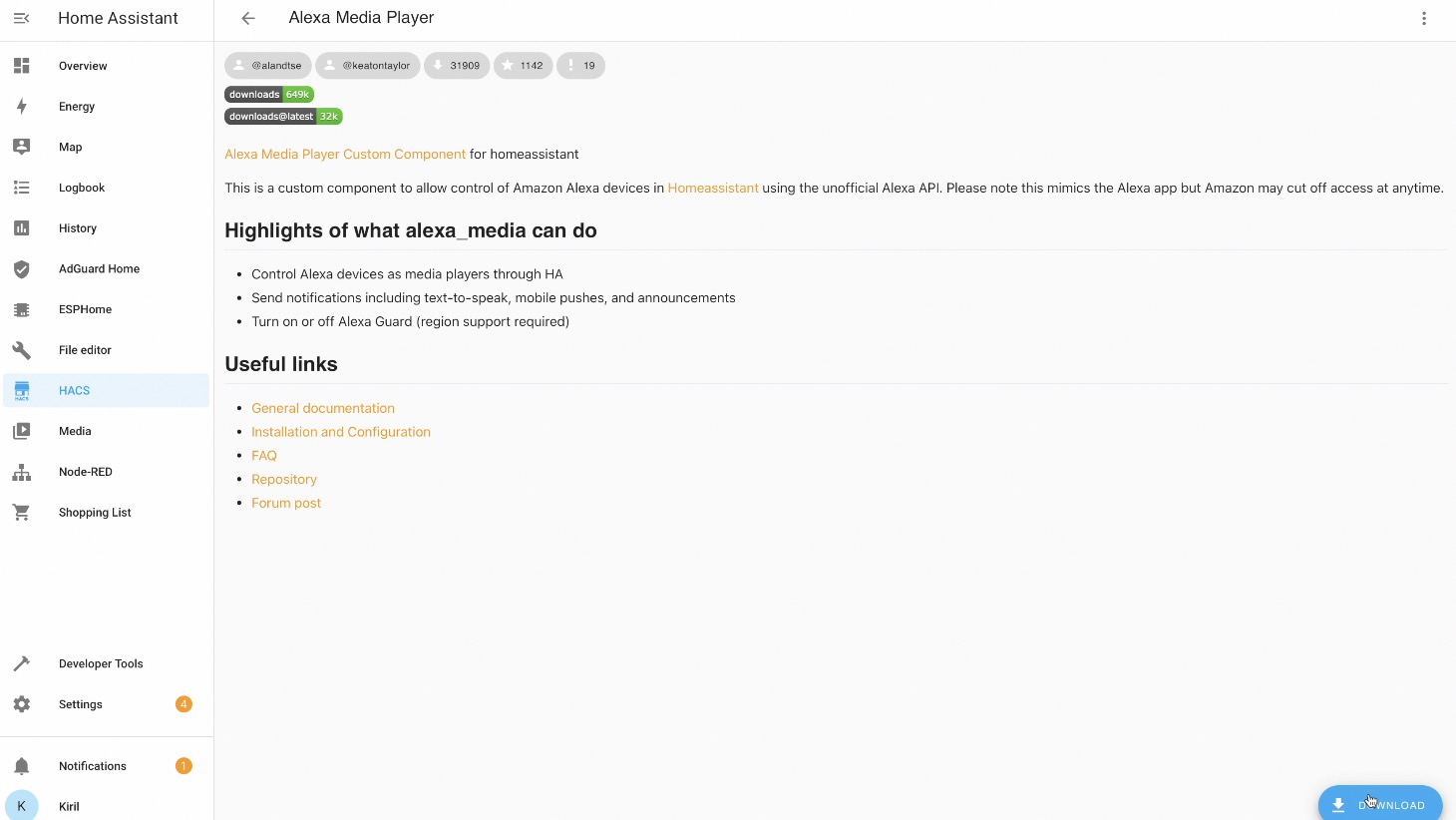This image showcases a screenshot from an Amazon-related website with two main sections: a narrow, vertical column on the left and a broader, off-white area occupying the rest of the page. 

**Left Vertical Column:**
- The left sidebar is largely white, featuring the heading "Home Assistant" in grey.
- Below this heading is a menu with grey icons, listing the following options:
  1. Overview
  2. Energy
  3. Map
  4. Logbook
  5. History
  6. AdGuard Home
  7. ESPHome
  8. File Editor

- The "HACS" option is highlighted in bold with a blue background.
- Continuing down the list are:
  9. Media
  10. Node-RED
  11. Shopping List
  12. Developer Tools
  13. Settings

- Below the settings, there's an orange icon with a white "4" and another orange icon with a white "1" indicating notifications.
- The bottom section reads "CIRL" in black letters next to a blue icon with a capital "K."

**Main Content Area:**
- The center section features a grey back arrow in the top-left corner.
- To the right of the arrow, the title "Alexa Media Player" is in black lettering.

**Button and Information Area:**
- Below the title, there are five rectangular grey buttons labeled as follows:
  1. Alendize
  2. Alendice
  3. @Keaton Taylor
  4. 31909
  5. 1142
  6. 19

- Further down are two sets of two-tone rectangular bars:
  1. First set labeled "Downloads" with "649K" on the right.
  2. Second set labeled "Downloads (latest)" with "32K" on the right.

- An orange-highlighted section reads "Alexa Media Player Custom Component for Home Assistant."
- Below it is a bolded paragraph title "Highlights of what Alexa Media can do" followed by three bullet-pointed items.

**Useful Links Section:**
- The "Useful Links" heading is in bold, followed by five bullet points with orange text on the right:
  1. General Documentation
  2. Installation and Configuration
  3. FAQ
  4. Repository
  5. Forum Post

**Download Button:**
- In the bottom-right corner is a blue oval button with "Download" and a white down arrow.

Overall, this image showcases a detailed interface for managing various components related to Amazon's home automation services using the Alexa Media Player, along with download metrics and useful documentation links.